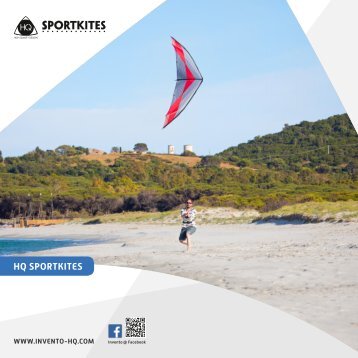In the center of this advertisement image, a woman is captured flying a kite on a beach. The photograph, predominantly set against a backdrop of blue skies, white clouds, and lush greenery, emphasizes the serene and expansive environment. Above her, a vibrant kite decorated in shades of gray and red contrasts with the sky, trailing down to her grasp on the sandy shore. The beach appears tranquil and almost deserted, with only a small body of water visible to the left and buildings faintly discernible in the distance, obscured by the foreground hills and trees.

Text elements frame the visual scene: in the upper left corner, set against a white background, the words "HQ Sport Kites" are prominently displayed in black. The same text appears centrally at the bottom of the image, alongside the website URL "www.invento-hq.com" and small icons for Facebook and another symbol. The overall composition, marked by the stylistic placement of text and images, unmistakably conveys the format and style of an advertisement, crafted to draw attention to the kite and its brand.